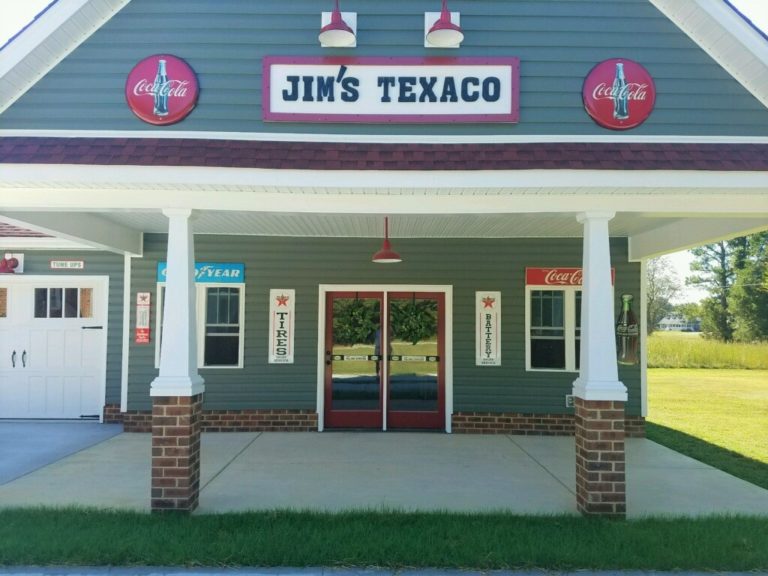This image captures the storefront of Jim's Texaco, a hybrid general store and gas station that also appears to function as an auto body shop. The building prominently features a sign that reads "Jim's Texaco" in dark navy blue letters against a white rectangular background trimmed in red. Flanking this sign are two circular Coca-Cola advertisements, each displaying the iconic red dot, bottle, and white script logo of Coca-Cola. Illuminating the sign from above are two mounted lights.

The structure itself is composed of both brick and wood, with the brick forming the lower portion and sturdy pillars that support the wood-paneled upper section and the triangular roof. The facade includes two large, red-bordered double doors with reflective coating, flanked by signage indicating services offered: one says "tires" and the other "battery."

Adjacent to these doors are two windows; one is branded with the Goodyear logo, while the other displays another Coca-Cola advertisement. To the left of the main entrance, there appears to be either one or two garage doors equipped with vehicle lifts, underscoring the store's function as an automotive service provider.

In the foreground, a strip of grass abuts the sidewalk leading to the entrance, while the background features trees and taller grass, adding a touch of rural charm to the scene.